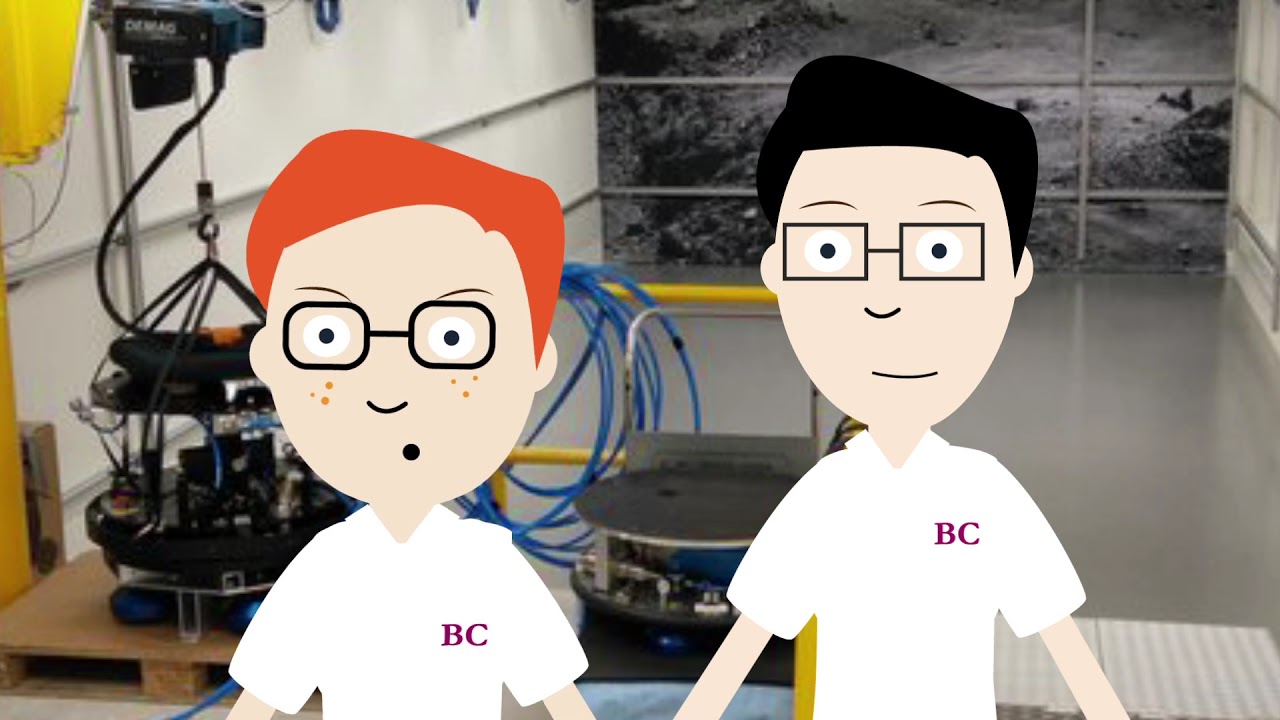In this wide rectangular image, two cartoon characters stand centrally in front of a real-life scene that appears to be set in a high-tech robotics studio. Both characters have white skin and wear glasses, sporting white shirts adorned with the letters ‘BC’ in red. The character on the right has black hair and square glasses, while the character on the left has red hair, square glasses, and orange freckles. They gaze directly at the camera, set against a backdrop that combines various elements of a scientific or technological environment. 

The floor of the studio is gray and shiny, leading to a wall at the back, which is visible in the top right corner and detailed with gray bars. This wall features a black-and-white photograph resembling an outdoor surface, potentially evoking a Martian or space-like landscape. Adjacent to this is a white wall, similarly barred in gray. Prominently, a yellow metal object stands near the center of the image, flanked by a large black robotic contraption on the left, replete with cylindrical components and various intricate elements. The presence of diverse tools, wires, and a mixture of colors including brown, white, purple, orange, tan, yellow, black, and gray bolster the impression of a sophisticated scientific setting, likely indoors within a science facility.